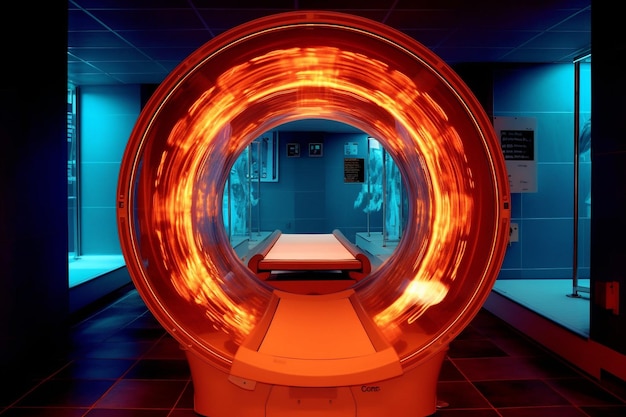The image depicts a dimly-lit room with a medical diagnostic machine prominently featured in the center. The machine resembles an open MRI scanner or similar equipment, characterized by a glowing, yellowish-orange circular ring mounted on a white base. Illuminating the room, the orange light emanates from the center of the circular ring, creating a striking visual focus. Directly behind the ring, a white platform or bed can be seen, suggesting the area where a patient would lie during a scan. The room itself has blue-colored walls with a modern, tiled design. The right side of the room contains a white box and various indistinct objects, possibly part of the medical setup or control units. Additionally, blue ambient lighting or possibly smoke hints at a sterile, high-tech atmosphere. The floor is adorned with square tiles, adding to the clinical environment.